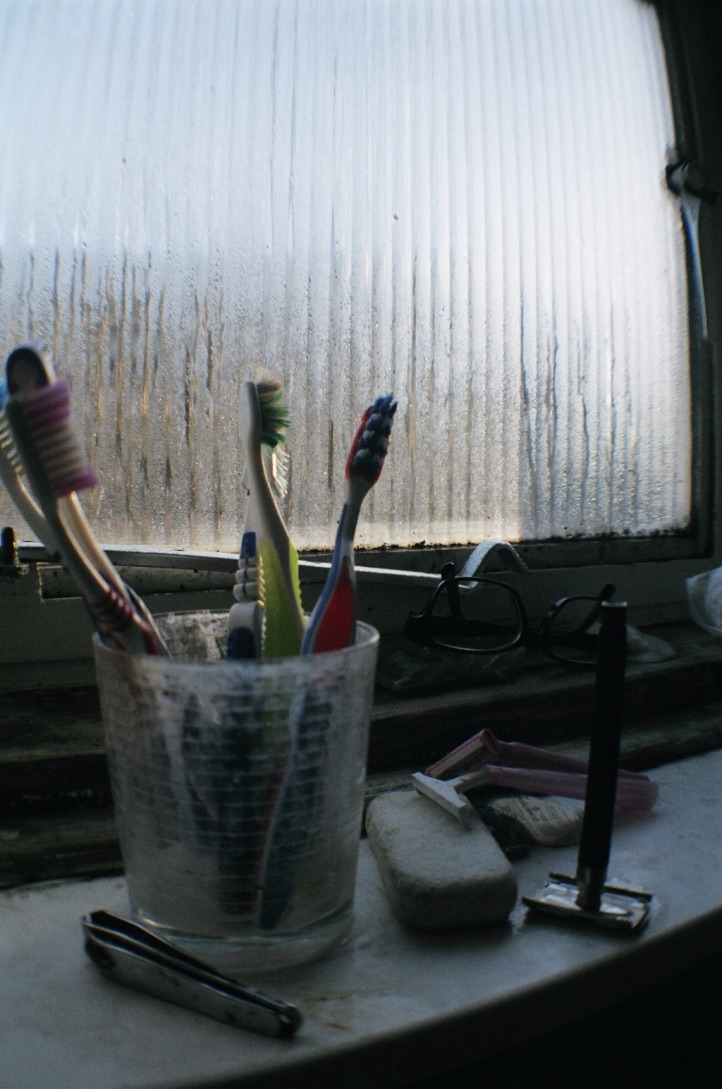A close-up, color photograph captures a cluttered bathroom windowsill or vanity shelf in soft, shadowy light, likely taken on a smartphone. At the center, a clear glass cup, streaked with scum marks from water and toothpaste, holds five upright toothbrushes. To the cup's left lies a stainless steel nail clipper, collapsed with its handle oriented downward. On the right, a bar of traditional soap hosts a women's razor, identifiable by its pink handle and white head, resting blade-down atop the soap. Nearby, another razor stands with its blade down on the shelf. In the background, a slightly opaque window with vertical ribbed lines offers limited visibility, hinting at outdoor elements such as trees with a brownish detail at the lower third. A metal clasp for opening and locking the window is visible at the bottom. The overall image is dimly lit, with sunlight streaming through the translucent window, casting a faint shadow over the assortment of personal hygiene items. No text or additional markings are present in the photograph.